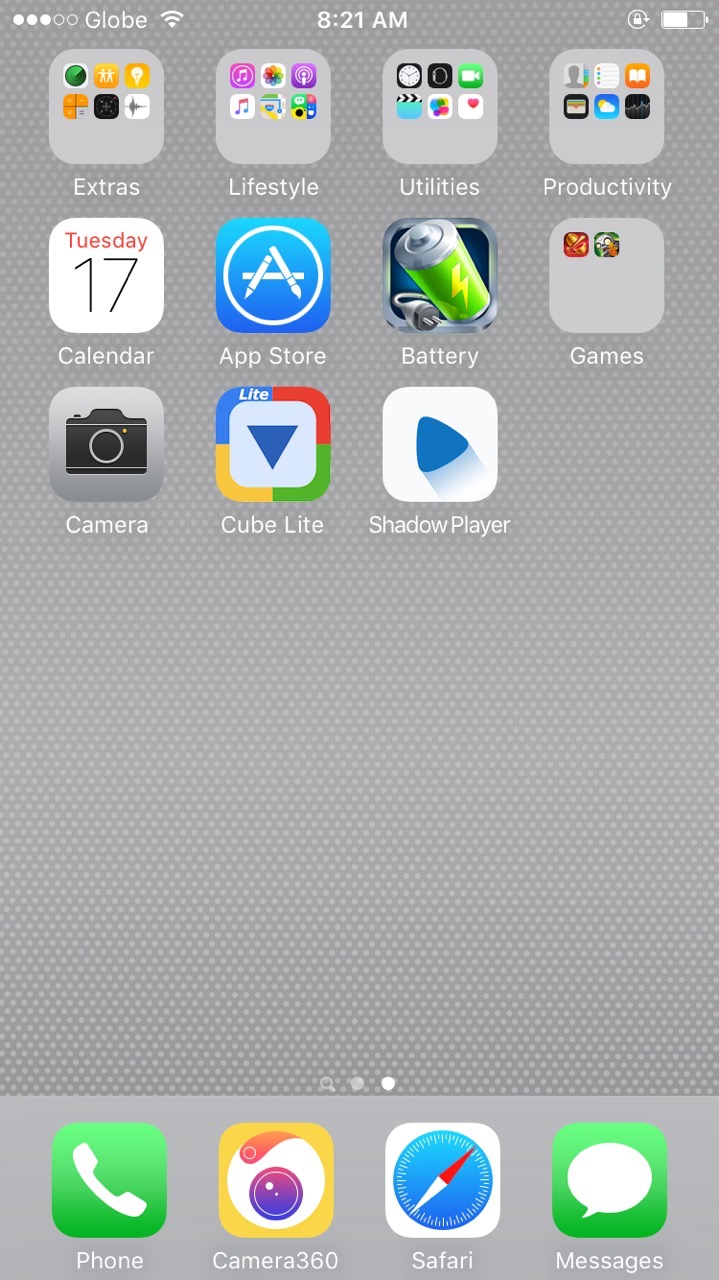The image is a detailed screenshot of an iPhone home screen. The background features a medium glow color with lighter gray dots scattered across it, creating a subtle, textured effect. In the upper left corner, the carrier name is visible as "Globe" along with the Wi-Fi symbol, indicating an active connection. The time displayed in the center of the screen reads 8:21 a.m. In the upper right corner, the battery icon shows approximately two-thirds charge.

The screen showcases various app icons, many of which are organized into categories. The visible categories include "Extras," "Lifestyle," "Utilities," "Productivity," and "Games," each containing multiple app icons. In addition to the categorized apps, several standalone apps are also visible, comprising "Battery," "App Store," "Calendar" (indicating it is Tuesday the 17th), "Camera," "Cube," "Light," and "Shadow Player."

Towards the bottom of the screen, icons for the iPhone's default apps are positioned for quick access. These include "Phone," "Safari," "Messages," and the "Camera 360" app. The screen layout appears well-organized, balancing both productivity and entertainment applications.